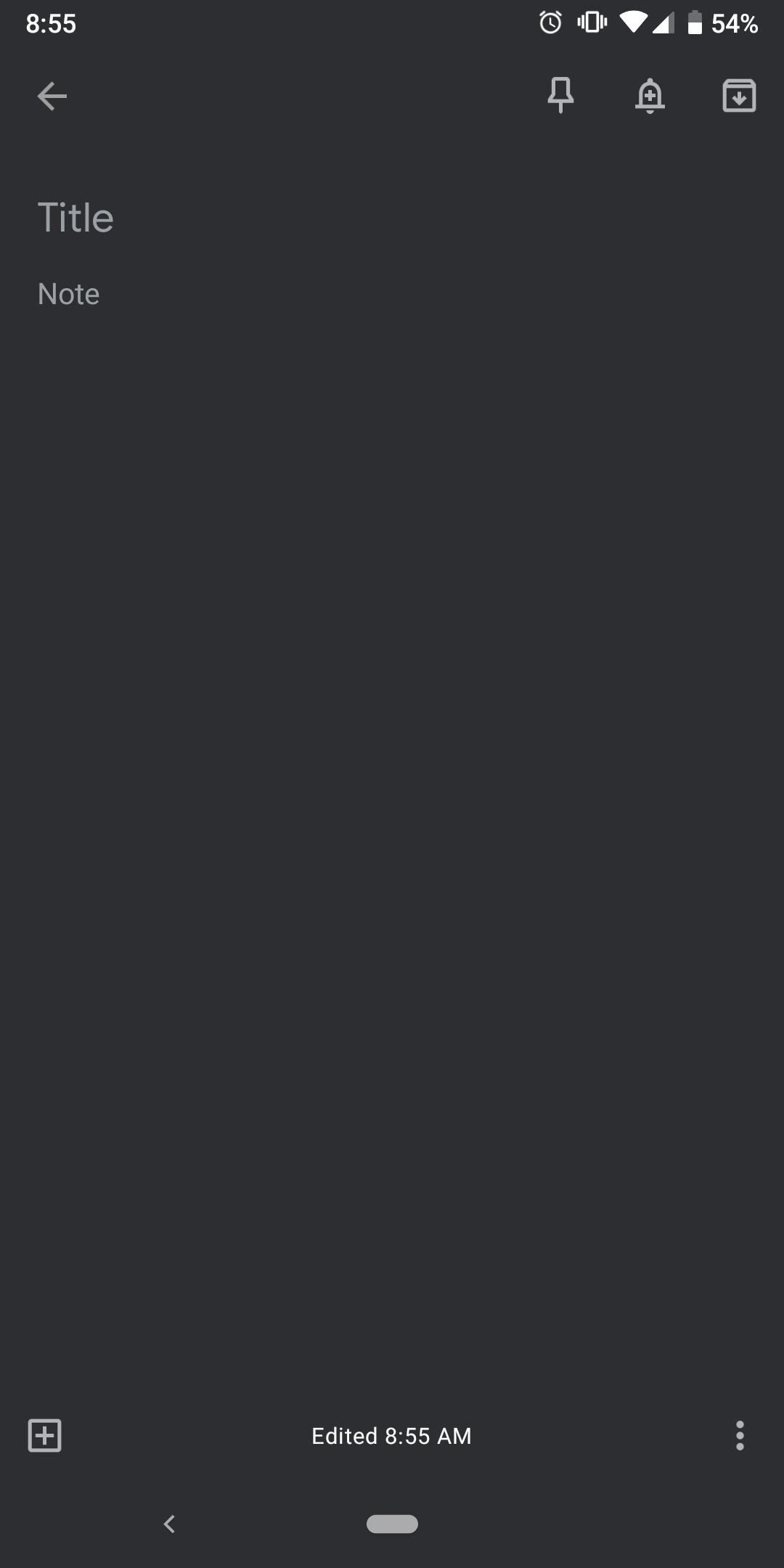This image is a screenshot from a mobile device, though the operating system (Android or iOS) is not specified. The screen has a dark grey background, including the status bar which is the same dark grey color. The time displayed is 8:55 AM. In the status bar, there are icons indicating an active alarm, vibration mode, WiFi connectivity, cellular signal strength, and a battery life of 54%.

Below the status bar, there are three action icons: a white pin icon, a bell icon, and a download icon represented by a file with a downward arrow. Under these icons, the text "Title" appears in grey, indicating an area to input the title of a note, followed by smaller grey text labeled "Note" for entering note content. This suggests that the screenshot is from a note-taking application designed for creating to-do lists or saving notes. The majority of the screen is blank, showing the dark grey background. At the bottom of the screen, it reads "Edited 8:55 AM," indicating the last time the note was modified.